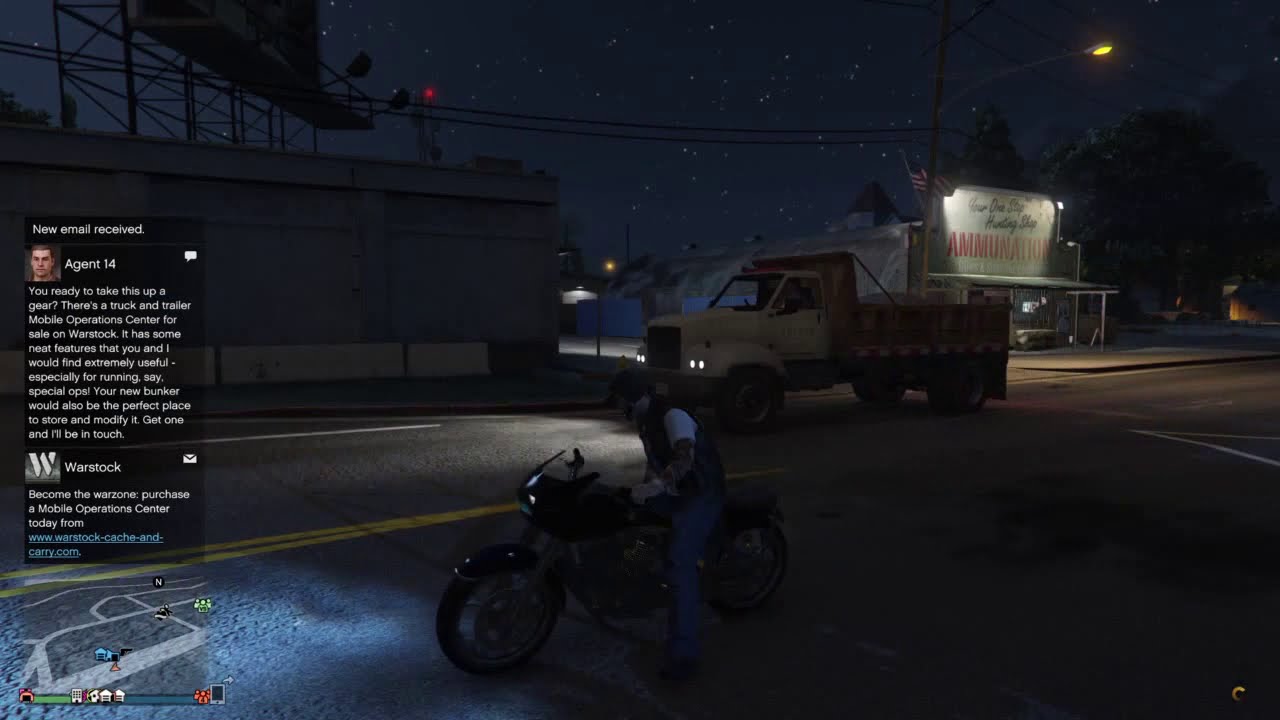This image, likely taken from an open-world video game reminiscent of Grand Theft Auto, captures a nighttime scene illuminated by a star-studded black sky. In the forefront, a paved asphalt street with a yellow dividing line runs horizontally. A man character is depicted sitting idle on a motorcycle, clad in a white t-shirt, black vest, blue jeans, and either a helmet or hat. Situated behind him in the adjacent lane is a beige utility truck with its headlights on, reflecting light off the road.

In the distance, you can discern streetlights, electrical wires crisscrossing the sky, and a prominent billboard on the left advertising "AMMUNition" in red letters above what appears to be an Americana-style grocery store. Additionally, a gray building with another billboard atop adds to the backdrop.

On the left side of the screen, a black-highlighted notification indicates a new email has been received from a character named Agent 14. The email reads: "You ready to take this up a gear? There’s a truck and trailer mobile operation center for sale on Warstock. It has some neat features that you and I would find extremely useful, especially for running, say, special ops. Your new bunker would also be the perfect place to store and modify it. Get one, and I’ll be in touch." Further down, the email is signed off with, "Become the Warzone. Purchase a mobile operation center today from www.warstock-cache-and-carry.com."